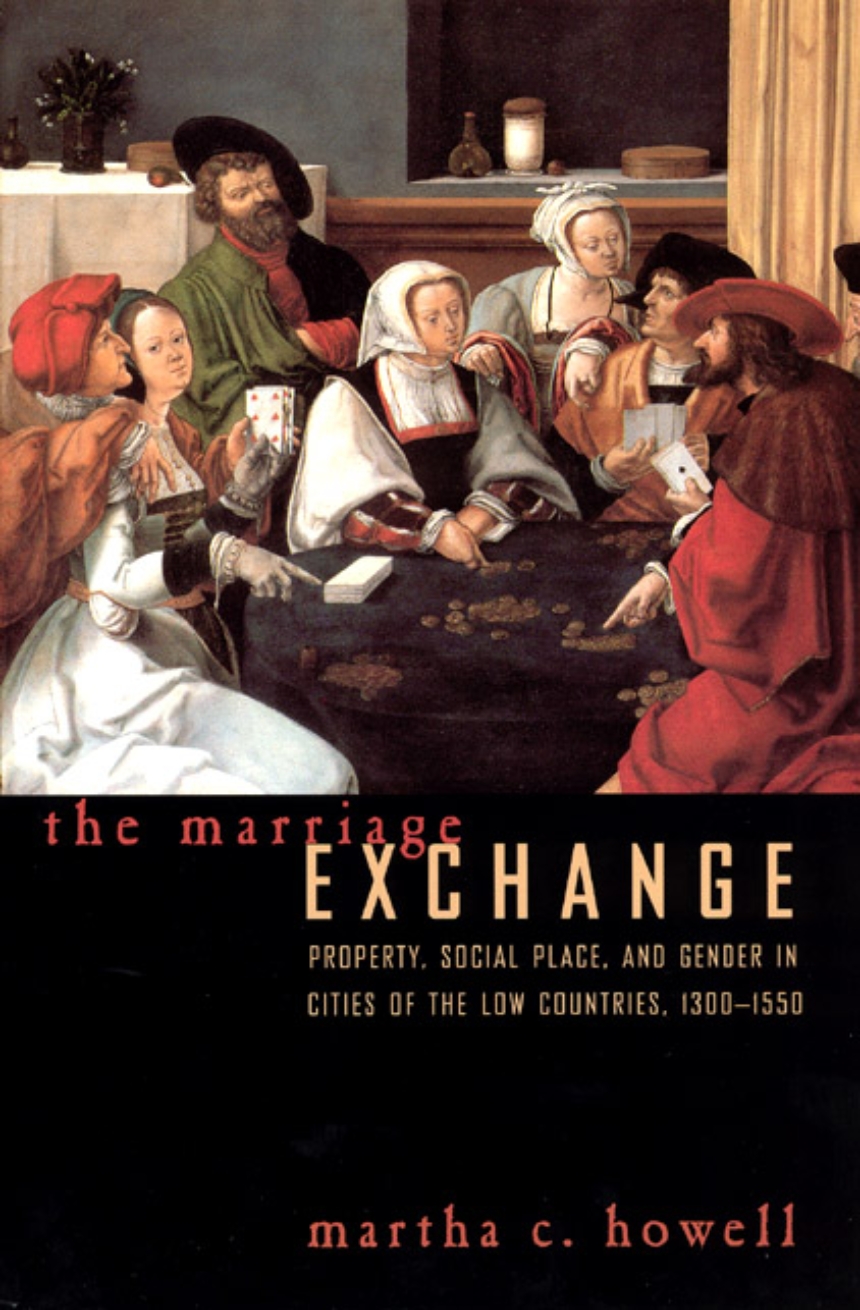The cover features a detailed illustration set in a medieval or ancient period. It depicts a group of men and women sitting around a round table draped with a purple cloth, playing cards. The men are attired in long cloaks and wide-brimmed hats, while the women are in gowns with scarves or headdresses covering their heads, some adorned with white gloves and jewelry. The setting is an interior room with a grayish-blue wall, brown curtains to the right, and a white tablecloth-covered table with a vase of white flowers on the left. Behind the players, an array of brown cabinets holds various food items, plates, a jar, and a lit candle. The individuals appear engrossed in their game, holding and examining white poker cards, surrounded by scattered brass-colored coins. Below the illustration, the text reads, "The Marriage Exchange: Property, Social Place, and Gender in Cities of the Low Countries 1300-1550" in uppercase letters with a sans-serif font, while "Martha C. Howell" is written at the bottom in red, serif font on a black background.